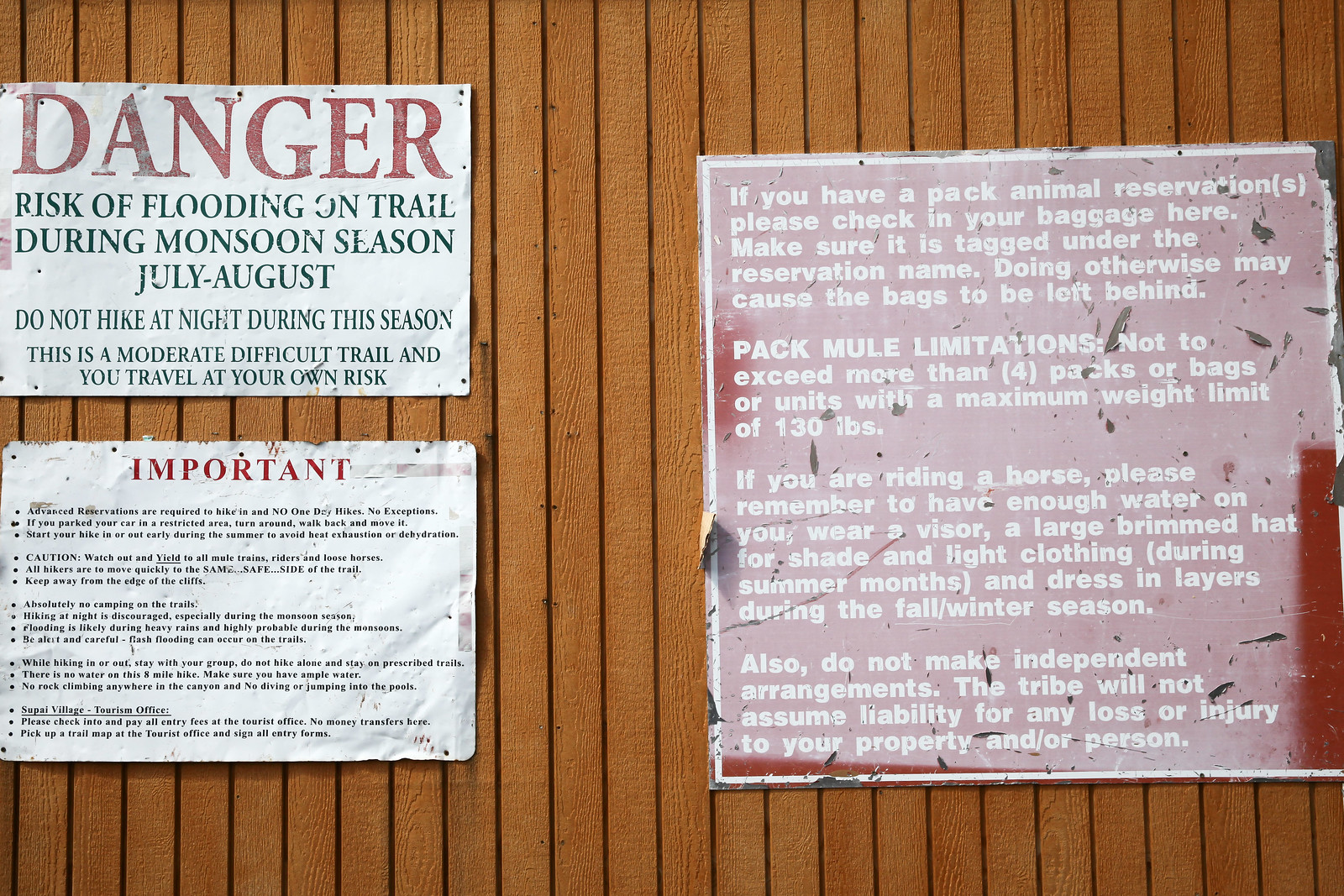The image depicts a wall clad in vertical wooden planks, to which three distinct signs are affixed. On the left side, two white signs with red and black text are positioned one above the other. The top sign reads, "Danger! Risk of flooding on trail during monsoon season, July to August. Do not hike at night during this season. This is a moderately difficult trail and you travel at your own risk." Below this, a sign with a red header labeled "Important" presents a series of bullet points with safety instructions in very small print, which are hard to read. On the right-hand side of the wall, there is a red sign with white text indicating, "If you have a pack animal reservation, please check in your baggage here. Make sure it is tagged under the reservation name. Doing otherwise may cause the bags to be left behind." Additional instructions outline, "Pack mule limitations: not to exceed more than four packs or bags or units with a maximum weight limit of 130 pounds. If you're riding a horse, remember to have enough water, wear a visor or large-brimmed hat for shade, and light clothing during summer. Dress in layers during fall and winter. Also, do not make independent arrangements. The tribe will not assume liability for any loss or injury to property and/or person."